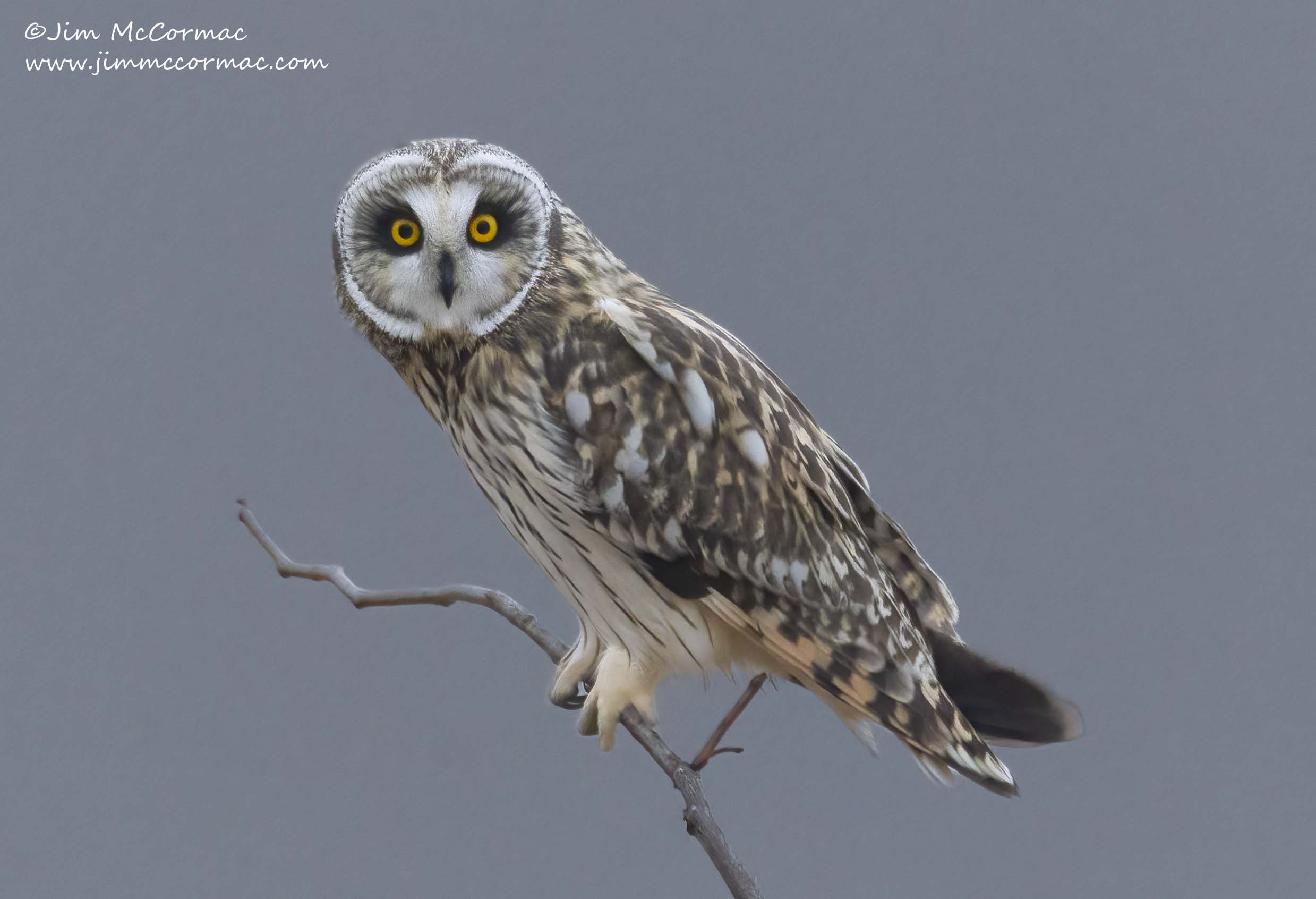The image captures a striking owl perched on a protruding brown twig, gazing directly at the camera. The owl's vivid golden eyes, deeply set against a background of black and gray feathers, stand out prominently. Its face is predominantly white, accentuated by faint gray lines that outline the facial features. The owl's plumage is a harmonious blend of brown, gray, and white, with a predominantly white breast adorned with specks and streaks of gray and black. The entire scene is set against a uniform gray backdrop, lending a stark contrast that highlights the owl's detailed markings. At the top left corner, the image credits Jim McCormick, with a copyright symbol and the website www.jimmccormick.com.